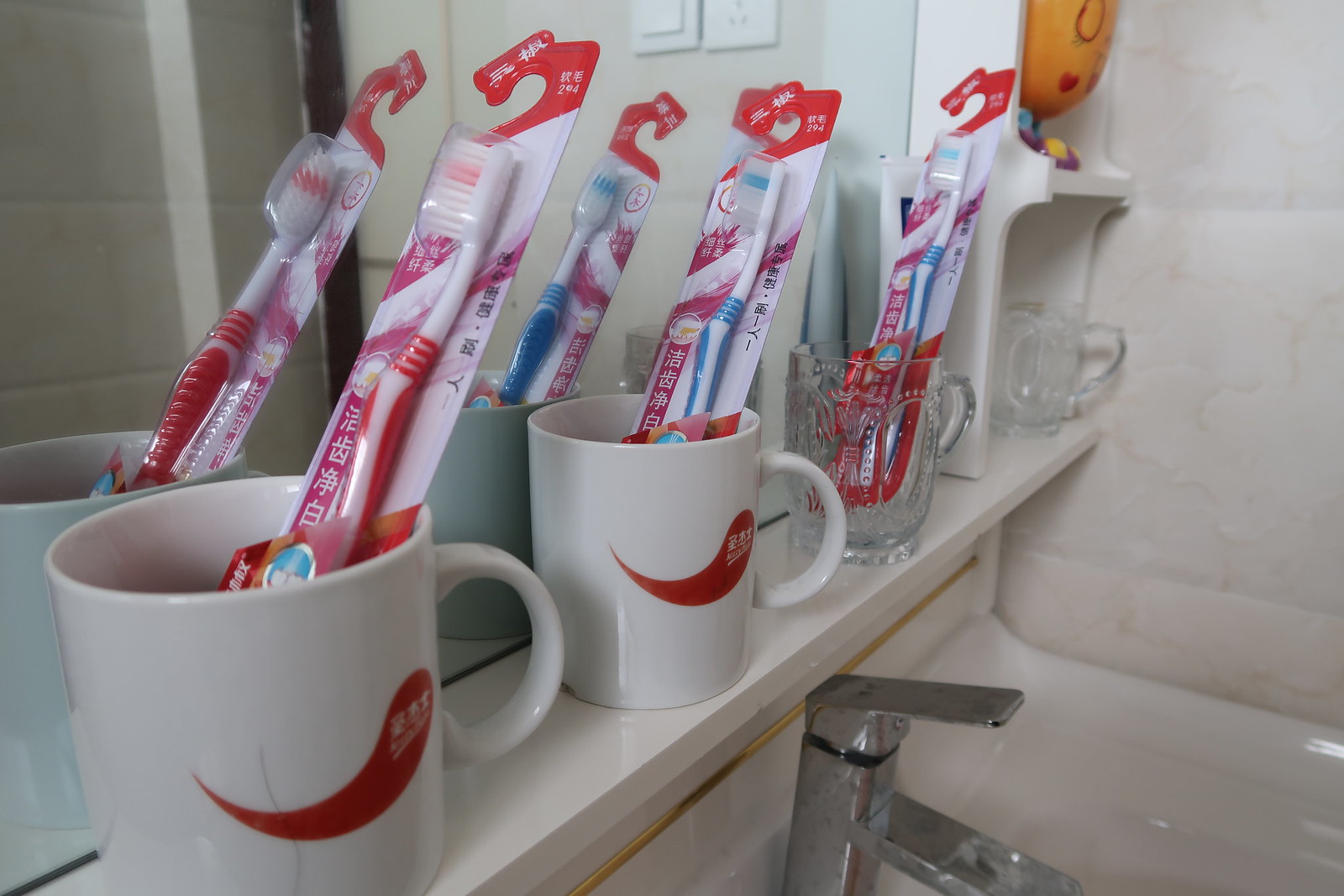This photograph captures a detailed view of a bathroom countertop arrangement. Predominantly, the white ceramic wall contains a mirror reflecting parts of the bathroom, situated above a white sink with a stainless steel faucet and handle. Affixed below the mirror, a small shelf holds four cups: two white ceramic coffee mugs each adorned with a red teardrop pattern, and two clear glass cups. Each of the two ceramic mugs contains a toothbrush still in its packaging; one featuring red and white bristles, the other blue and white bristles. One of the clear glass cups also holds a toothbrush with similar packaging, exhibiting Asian characters indicative of Japanese or Chinese origins, while the other clear glass cup remains empty. Additionally, a light switch and power socket can be seen near the left side of the mirror. Attention to detail extends to the cups on the shelf, highlighting the variety and distinctive packaging of the toothbrushes while emphasizing the neat and organized layout of the bathroom counter.